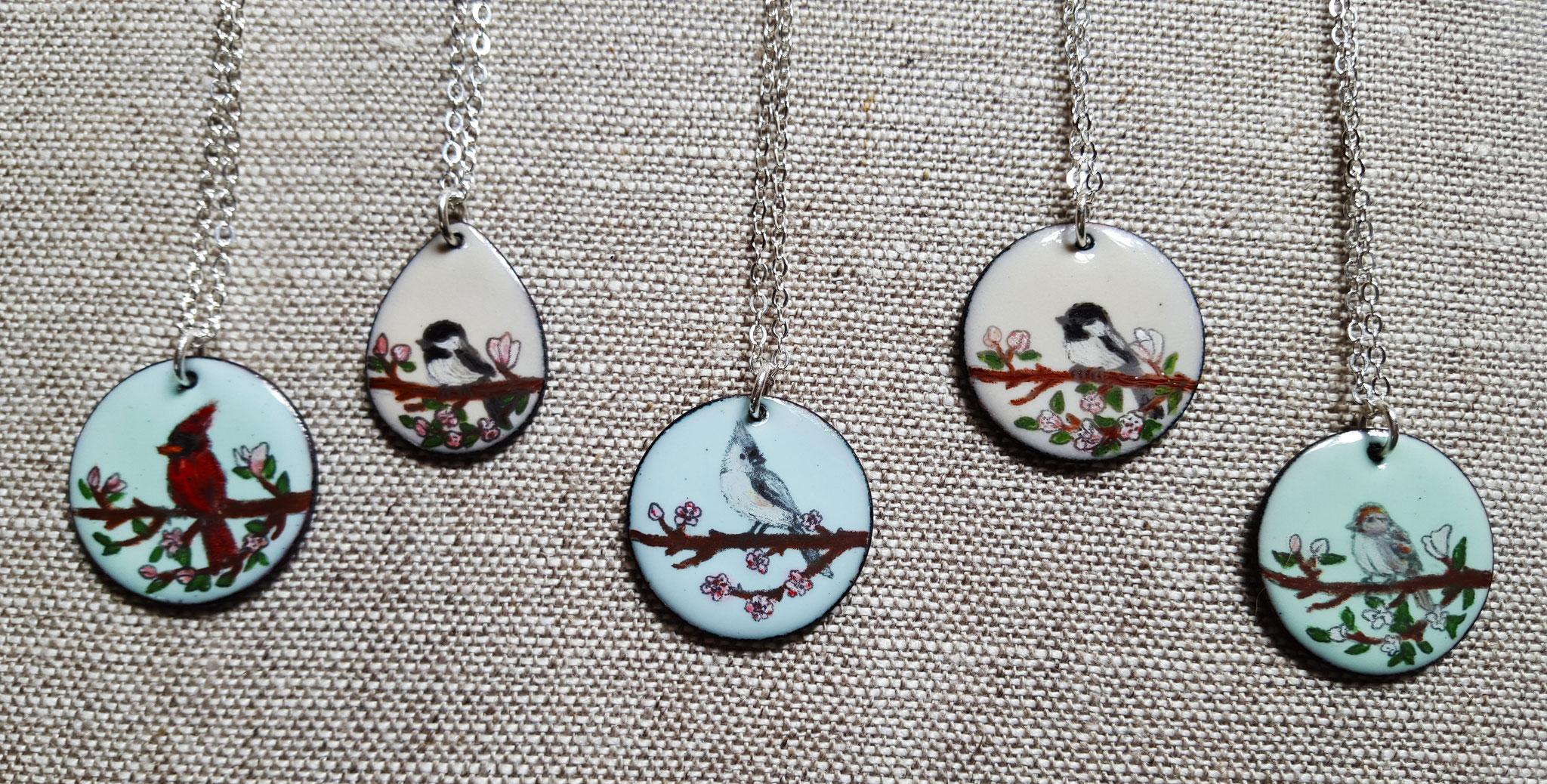This detailed photograph showcases five necklaces artfully arranged on a beige burlap fabric. Each necklace features a unique pendant charm, four of which are circular, and one is teardrop-shaped. The pendants are crafted from silver and hang from delicate silver chains. Each charm displays an illustration of a bird perched on a branch adorned with flowers. The backgrounds of the charms vary between white and pale pink, enhancing the vibrancy of the birds. The collection includes a striking red cardinal set against a blue background with cherry blossoms, a colorful blue jay among delicate blossoms, two charming images of chickadees, and an unidentified bird, all perched in scenic floral settings. The birds' vibrant colors stand out beautifully against their soft backgrounds, making each necklace a captivating piece of art.